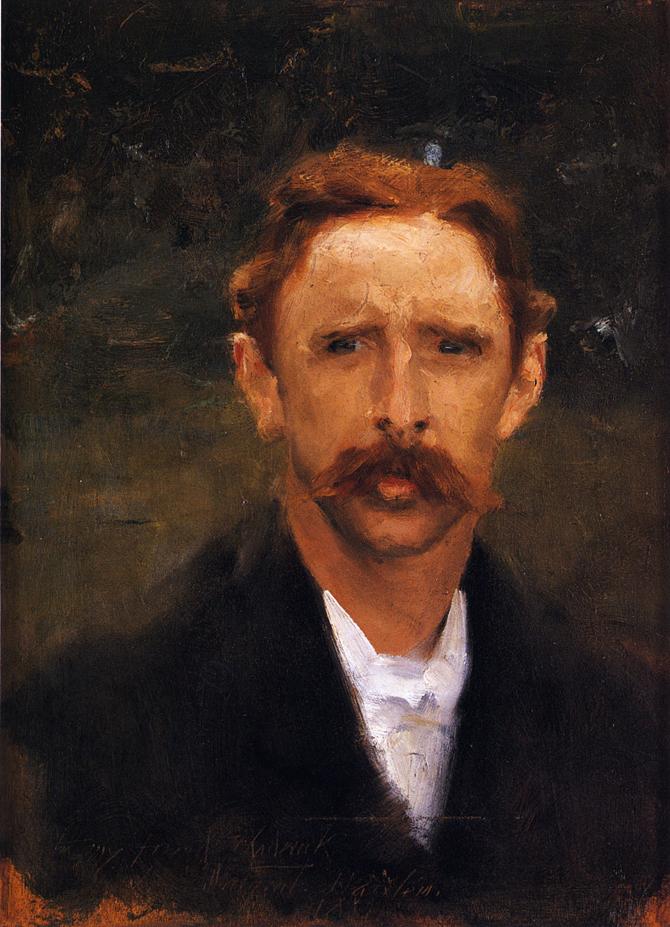This vertically aligned rectangular painting depicts a man from the chest up, positioned centrally against a dark, swirled background. The dominant colors in the background are black and brown, with black at the top blending into brown in the middle, accented by corners tinged with rust colors. The man, with his orangish-brown hair parted down the center, matching eyebrows, and a long, handlebar mustache of the same hue, gazes slightly to the left with a pensive expression. He is dressed in a black suit jacket over a white dress shirt, buttoned at the neck. His dark eyes and solemn look suggest a contemplative mood. The background's swirling patterns enhance the painting's depth, and fine, unreadable brown text at the bottom adds a subtle detail to the overall composition. The artwork, seemingly a hand-painted piece, evokes an 18th-century aesthetic and wouldn't be out of place in a museum or art show.